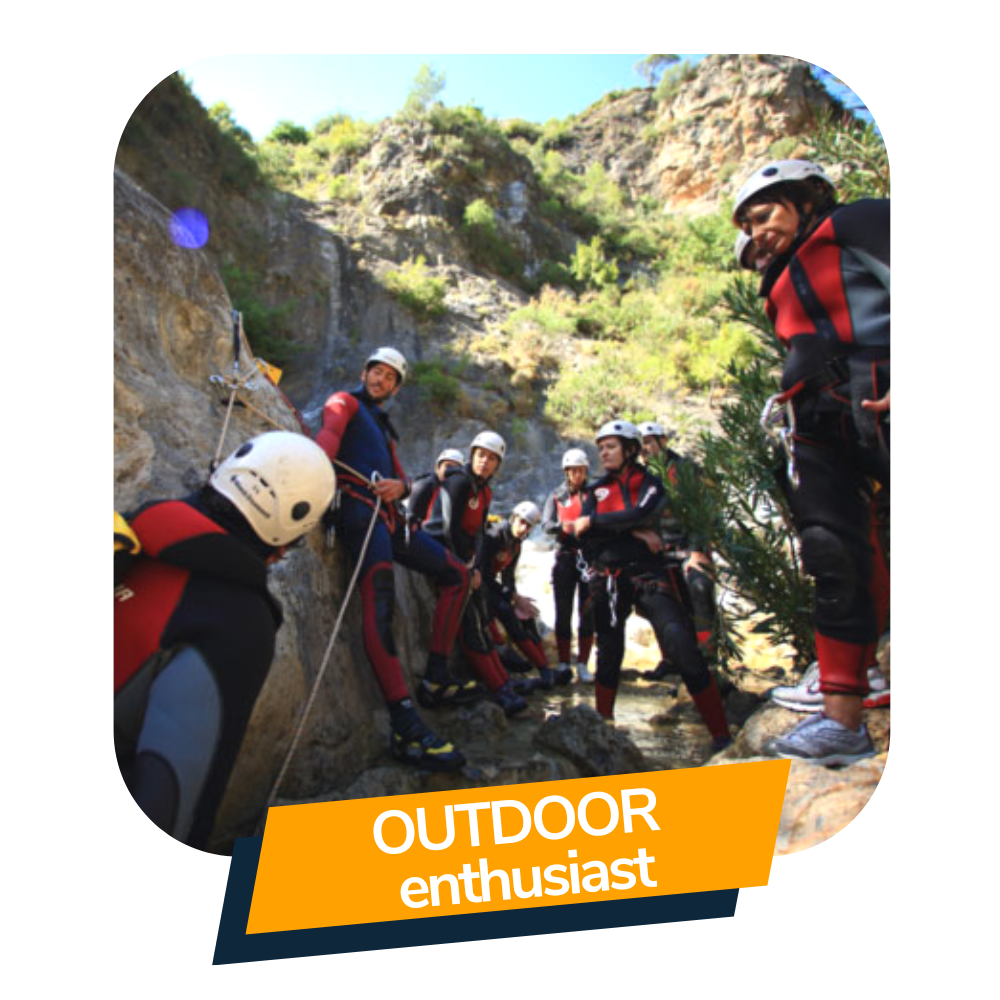The image features a group of approximately 10 individuals gathered in a rocky valley, surrounded by mountainous terrain lush with grass, trees, and bushes. They are all clad in matching outfits resembling wetsuits with red legs and arms and a blue bodice. Each person is equipped with white hard hats, backpacks, and various climbing gear. A rope is visibly attached to one member, suggesting he may have just completed a climb. The group appears focused on this individual, who seems to be the leader or the climbing guide. At the bottom of the photograph, an orange stripe with white lettering reads "Outdoor Enthusiast," hinting that this may be an advertisement aimed at adventure seekers and nature lovers.